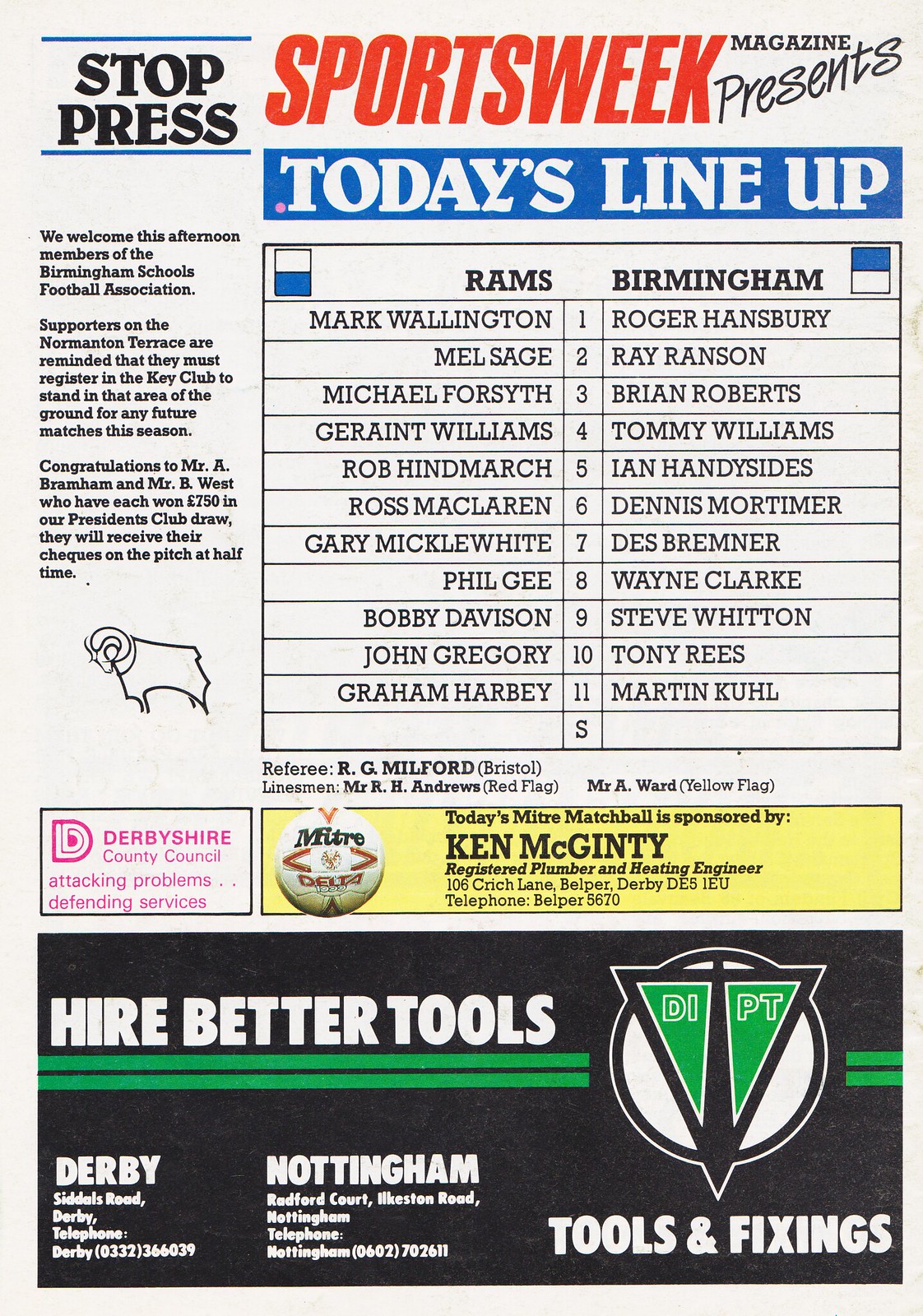The image appears to be a scan from a magazine or sports program, specifically from "Sports Week" magazine. At the top of the page, the title "SPORTS WEEK" is prominently displayed in red, all caps, shifted slightly to the right. Below it, "MAGAZINE PRESENTS" followed by "TODAY’S LINEUP" in large white all-caps text stands out against a blue background.

The central section of the page lists the lineup of two football teams: the Rams and Birmingham. The players' names are organized in two columns—Rams on the left and Birmingham on the right—each name in black all-caps text on a white background. The lineup includes:

1. Mark Wallington (Rams) vs. Roger Hansbury (Birmingham)
2. Mel Sage (Rams) vs. Ray Ranson (Birmingham)
3. Michael Forsyth (Rams) vs. Brian Roberts (Birmingham)
4. Geraint Williams (Rams) vs. Tommy Williams (Birmingham)
5. Rob Hindmarch (Rams) vs. Ian Handysides (Birmingham)
6. Ross MacLaren (Rams) vs. Dennis Mortimer (Birmingham)
7. Gary Micklewhite (Rams) vs. Des Bremner (Birmingham)
8. Phil Gee (Rams) vs. Wayne Clarke (Birmingham)
9. Bobby Davison (Rams) vs. Steve Whitton (Birmingham)
10. John Gregory (Rams) vs. Tony Rees (Birmingham)
11. Graham Harbey (Rams) vs. Martin Coolen (Birmingham)

An additional slot labeled “S” seems to be reserved for substitutes.

In the upper left corner, "STOP PRESS" is displayed in bold black font, followed by a welcoming message to the members of the Birmingham Schools Football Association and a reminder for supporters on the Normanton Terrace about Key Club registration requirements for future matches. Also mentioned is a congratulations note to Mr. A. Bramham and Mr. B. West, winners of £750 in the President’s Club draw, who will receive their checks on the pitch at halftime.

Below the lineup listings, the officials are listed: Referee R.J. Milford (Bristol), Linesman Mr. R.H. Andrews (Red Flag), and Mr. A. Ward (Yellow Flag).

The bottom third of the page is populated with advertisements. One in pink text promotes the Derbyshire County Council. Another yellow ad with a Mitre Delta soccer ball states that the match ball is sponsored by Ken McGinty, registered plumber and heating engineer (106 Critch Lane, Belper, Derby, DE5 1EEU, telephone Belper 5670).

At the very bottom, a large black and green advertisement for "Hire Better Tools" (DIPT is the company) includes the company’s logo of an upside-down triangle and details for their locations in Derby (Siddles Road, telephone 0332 366039) and Nottingham (Radford Court, Ilkeston Road, telephone 0602 702611). The ad emphasizes tools and fixings with all text in white.